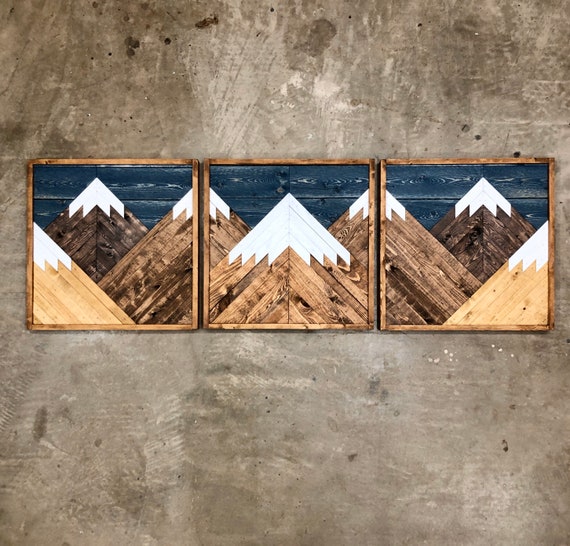The image showcases an artist's artwork consisting of three square frames, each framed with wood and arranged in the center against a textured, stone-like background with a blend of light brown, dark brown, and gray tones. The frames depict a continuous mountain range segmented across the triptych. The outer frames are mirror images, each featuring a composition of three mountains: a tan and white mountain on the outer edge, a black mountain with a white peak in the center, and a gray mountain with a white peak towards the center of the image. The middle frame presents the central gray mountain prominently with the adjacent mountains partially visible on either side, creating a cohesive scene. The sky is depicted with navy blue hues, emphasizing the peaks of the mountains. The overall effect is a harmonious overlap of triangular mountain tops, with the white peaks contrasting against the dark blue sky. No text is present in the image.